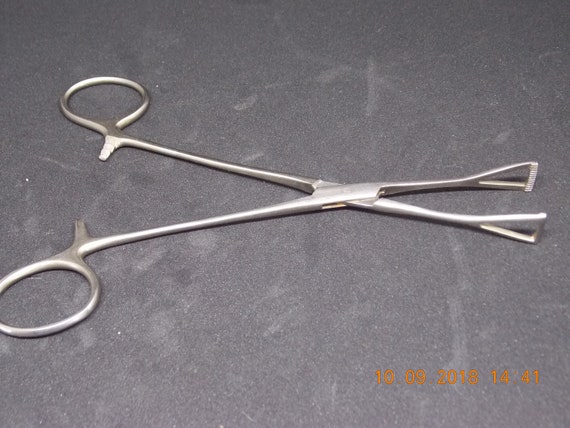The photograph is a close-up image capturing a pair of surgical forceps, likely made from stainless steel, given their silver color and reflective finish. The prongs, resembling a hybrid between scissors and tweezers, are shown in an open position, roughly halfway extended. The forceps rest on a notably scratched gray table, however, differing viewpoints suggest it could alternatively be a black table with a visible layer of dust, contributing to a disheveled appearance. In the bottom right corner of the image, the date "10.09.2018" and time "14:41" are displayed in a distinct orange font, dating the photograph to October 9, 2018, at 2:41 PM. The focus and positioning of the forceps suggest the photo is intended to document this medical tool, emphasizing their likely usage in a medical or clinical context.